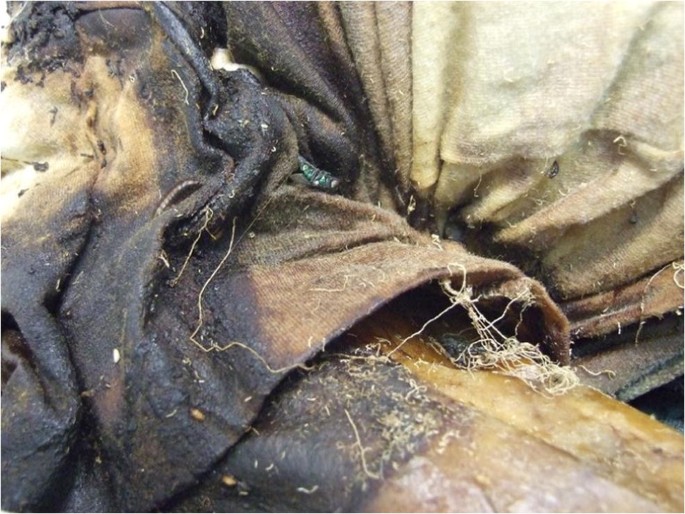The photograph presents a chaotic and intriguing assemblage of various items, each contributing to the overall complexity of the scene. In the upper left corner, there's a piece of clothing that appears to have been charred; the fabric is crumpled, blackened, and retains patches of tan or gray coloration amidst the predominant blackness. Moving to the upper right corner, more clothing is visible—this time, it's neatly folded and exhibits a cream color. Directly below this pile of clothing lies a piece of tile, distinguished by its dark brown hue. In the lower right corner of the image, a hard, beige-colored object draws attention. Its texture and appearance resemble rawhide, akin to what one might purchase from a pet store for a dog. This eclectic mix of elements renders the photograph a captivating study in texture and color contrasts.